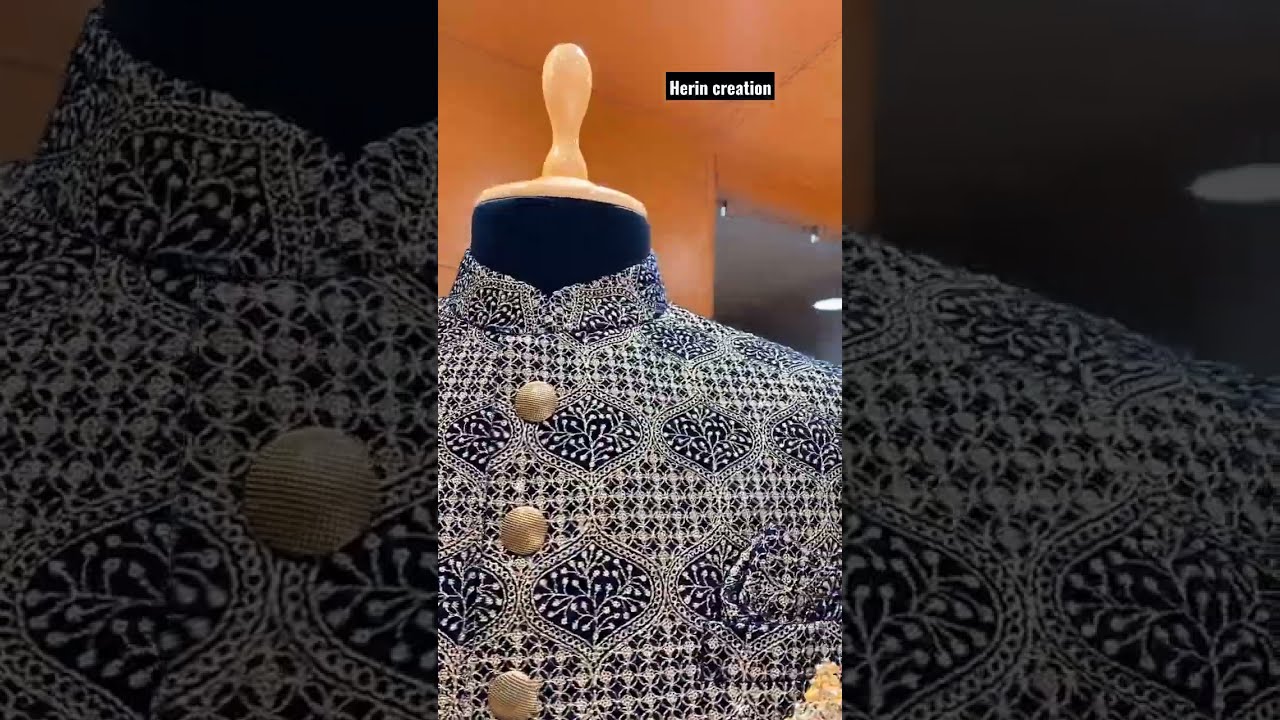The image depicts a detailed close-up of a high-collared blue and off-white tunic displayed on a headless wooden mannequin. The tunic features an intricate paisley pattern with three prominent goldish buttons running down the front. The background shows an orange wall and ceiling, with a black rectangular sign that reads "Heron Creation" in white lettering. The central focus is the clear, colored image of the tunic, flanked by sections of the same image that have been darkened and enlarged, showcasing the top neckline and shoulder parts. The tunic appears to be culturally influenced, possibly of Indian or Islamic origin. Additionally, the mannequin has a brass circular knob with horizontal lines on top where the head would be.